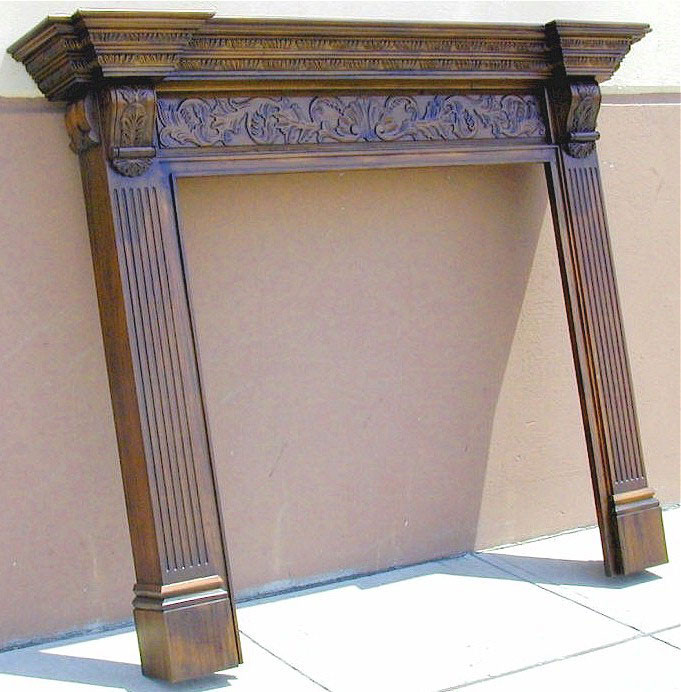This image captures a beautifully detailed wooden mantle, propped up against a pinkish-tan wall. The wall has a light colored upper section and a horizontal division, possibly made of wood, crossing the middle. Below this division, the wall resumes its tan hue. The floor is covered in large white tile, and the sunlight streaming in adds a bright reflection to the scene, suggesting it might be outdoors or in a well-lit area. The mantle, dark in color and made from a shiny wood, appears to have been removed from a fireplace and temporarily placed against the wall. Its design features intricate and artistic hand-carved decorations. The sides of the mantle showcase straight line designs, while the top is adorned with ornate leafy patterns and decorative etchings that reflect the high level of craftsmanship.